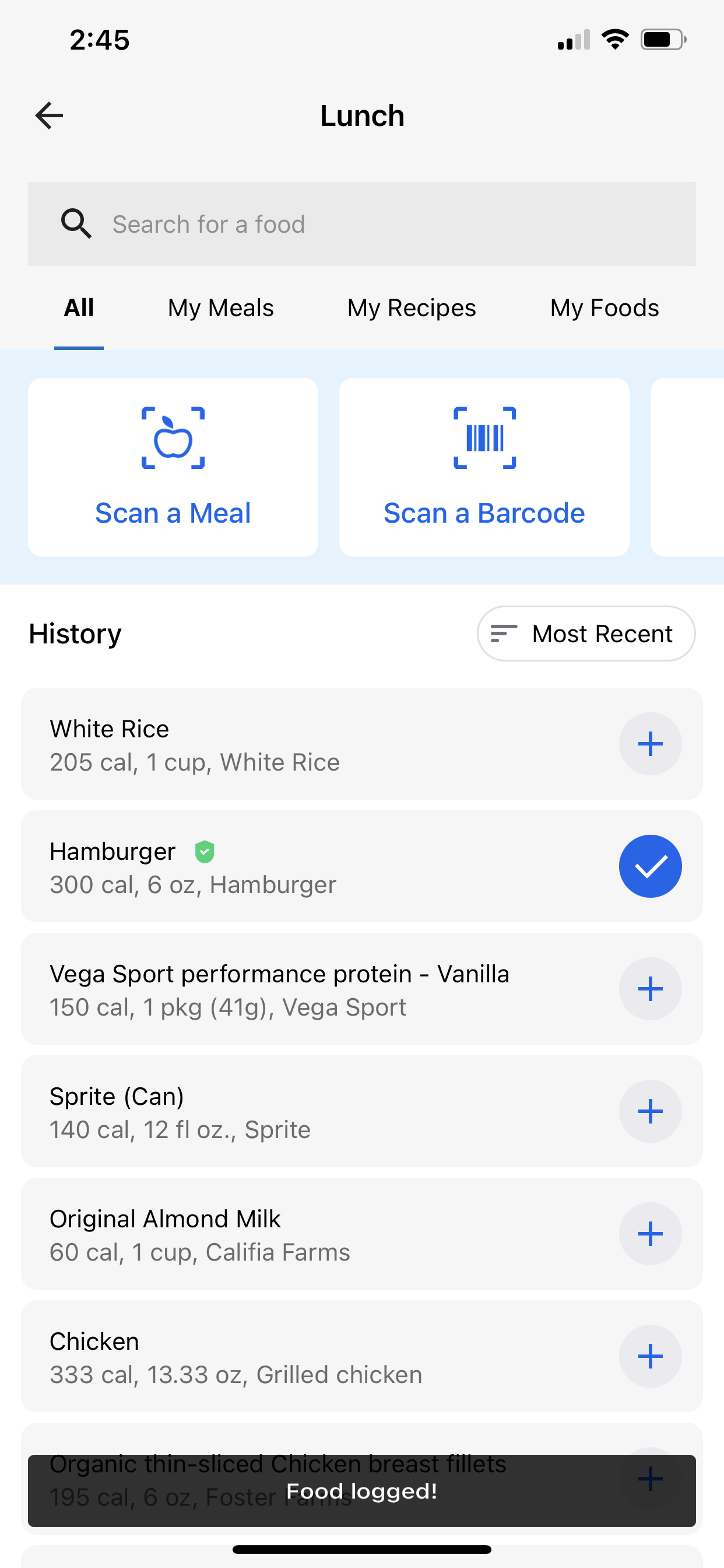Screenshot of a meal or calorie tracking app displays the "Lunch" option prominently at the top center of the screen, indicating it as the selected meal category. The top of the screenshot, which appears to be taken from a phone, shows the time on the left side, and reception, Wi-Fi, and battery icons on the right.

To the left of the word "Lunch," an arrow icon is visible, suggesting navigation back to a previous screen. Directly below this header, a light gray search box stands out against a predominantly white or light gray background; it contains the prompt "Search for a food."

Below the search box, four selectable categories are listed: "All My Meals," "My Recipes," and "My Foods." A light blue section beneath these options offers functionalities including "Scan a Meal" and "Scan a Barcode," with a partially obscured third option that requires scrolling to be revealed.

The subsequent section, with a white background, is labeled "History," with sorting options to the right, set to "Most Recent." This section displays foods recently logged by the user, such as "White Rice," including its calorie count, quantity, and an add button (plus sign) for easy logging. The user has selected the "Hamburger" entry, as indicated by a black box at the bottom of the screen that confirms "Food Logged."

This detailed visual capture provides a comprehensive glimpse into the workings and interface of the meal logging app, highlighting its user-friendly features and navigation elements.